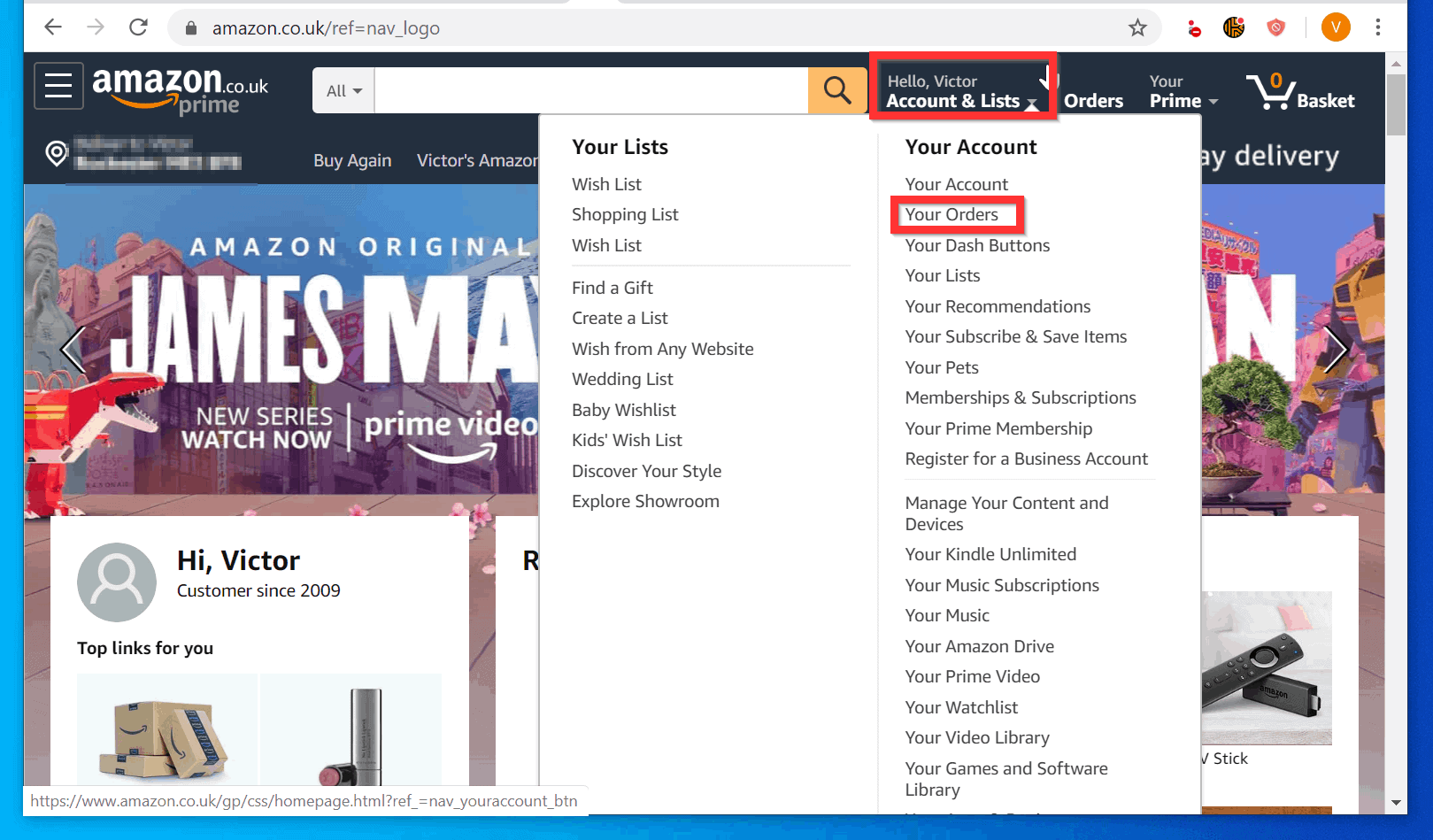**Detailed Caption for Amazon Homepage Screenshot:**

The screenshot depicts the Amazon homepage open to the amazon.co.uk website. At the very top, a gray search bar is prominently displayed, featuring a black padlock icon and the text "amazon.co.uk/ref=e_Nav_logo". Adjacent to the right side of this search bar, which has a pill shape, is a star icon, followed by four additional icons. The last icon is distinguished by an orange circle with three dots inside it. The browser window is outlined in blue, with a black top bar that displays "amazon.co.uk prime" on the left-hand side.

Below this, the Amazon search bar is visible, consisting of a departmental selection dropdown labeled "All," a white central area for text input, and an orange magnifying glass icon for search initiation. In the top line, a greeting "Hello, Victor" is noticeable, alongside "Accounts & Lists" highlighted in red, which opens a separate pop-up menu. This menu appears as a white pop-up containing various options for both user lists and account settings.

Dominating the main page background is a featured image promoting "Amazon Original James May: New Series - Watch Now on Prime Video." Beneath this promotional banner are three white boxes. The leftmost box greets the user with "Hi Victor, customer since 2009" and "Top links for you," displaying images of stacked Amazon brown boxes and a silver Stanley-style cup.

The pop-up menu on the top right contains two primary sections. Under "Your Lists" on the left, the categories include:
- Wish List
- Shopping List
- Wish List (repeated)
- Find a Gift
- Create a List
- Wish from Any Website
- Wedding List
- Baby Wish List
- Kids Wish List
- Discover Your Style
- Explore Showroom

On the right side, under "Your Account," the categories are:
- Your Account
- Your Orders (highlighted in red and selected)
- Your Dash Buttons
- Your Lists
- Your Recommendations
- Your Subscribe & Save Items
- Your Pets
- Memberships & Subscriptions
- Your Prime Membership
- Register for a Business Account
- Manage Your Content and Devices
- Your Kindle Unlimited
- Your Music Subscriptions
- Your Music
- Your Amazon Drive
- Your Prime Video
- Your Watchlist
- Your Video Library
- Your Games and Software Library

This detailed description encapsulates the various elements and layout of the Amazon homepage, highlighting the interactive components and user-specific features present on the screen.